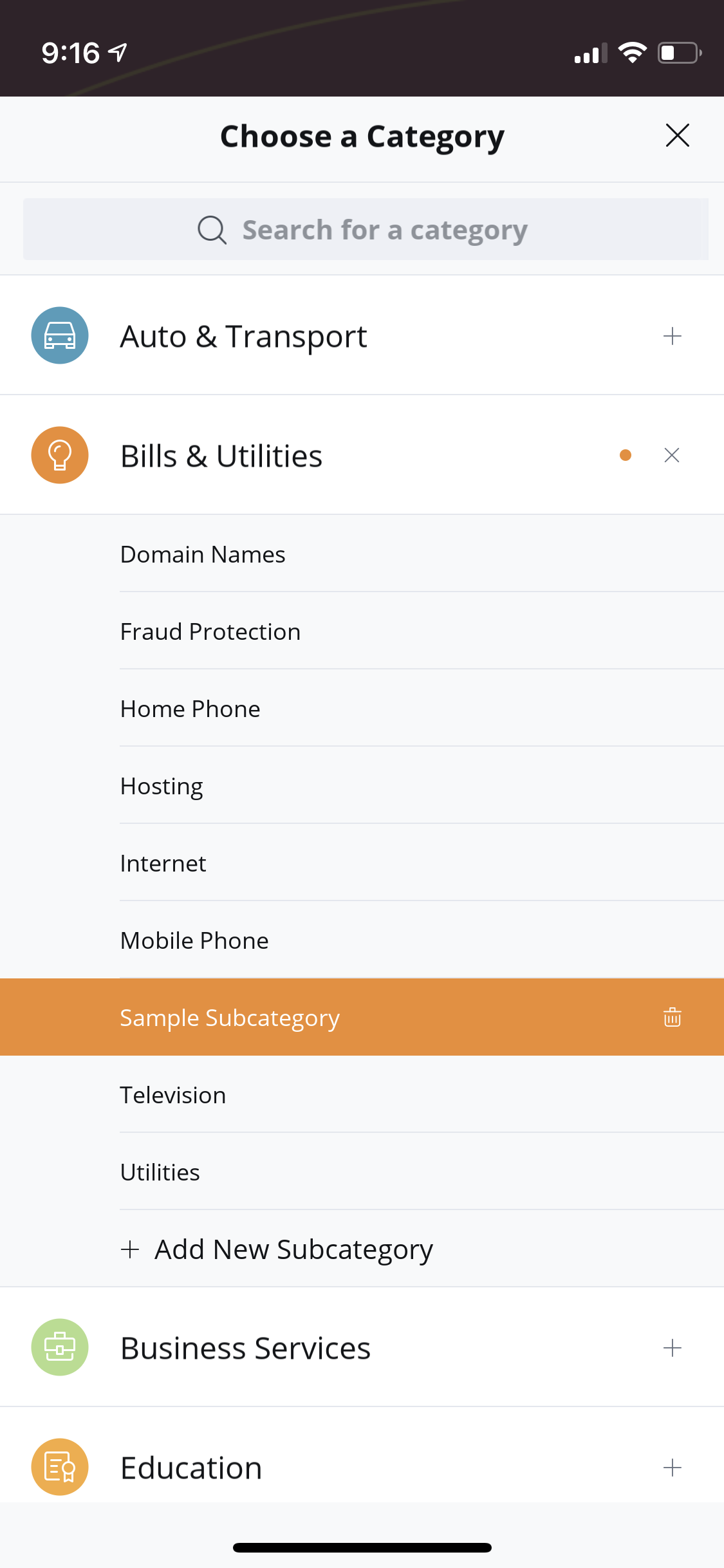A detailed screenshot from a mobile website displays various elements of a banking app. At the top of the screen, a black status bar shows the time as 9:16 with icons for Wi-Fi connectivity and signal strength, indicating the phone is online, while the battery icon shows approximately 25% remaining.

Immediately below, a white section features a prompt to "Choose a category" followed by a search bar labeled "Search for a category." The main content area starts with categories listed under "Auto and Transport," marked with a blue circle containing a small white car icon.

Next, "Bills and Utilities" is identified, accompanied on the right side by an orange circle with a light bulb icon. This category is expanded to reveal subcategories such as "Domain Names," "Fraud Protection," "Home Phone," "Hosting," "Internet," and "Mobile Phone," all in smaller indented text.

The following category is highlighted with an orange bar and white text reading "Sample Subcategory." Below this, subcategories like "Television," "Utilities," and an option to "Add New Subcategory" appear in black text.

Further down, "Business Services" is marked by a green dot with a white briefcase icon. Lastly, the category "Education" is identified by an orange circle with a diploma icon to the right side. 

A thin black bar runs across the bottom of the screen. This instructional screenshot, courtesy of First Hawaiian Bank, guides customers through the process of adding a subcategory to their banking system.